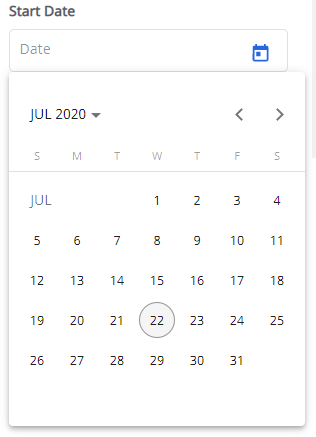**Caption:** 

A screenshot of someone's digital calendar is displayed on a clean, white background. The top corners of the calendar are accented with black sections. On the upper left, there's a label reading "Start Date." Below this, there's a small tab outlined in gray, which also contains the word "Date" on the left and an icon of a blue calendar on the right, with a generically highlighted date.

Overlaying this is a more prominent white calendar for July 2020. At the top, the month and year are indicated along with a drop-down arrow beside them. Navigation arrows are present on the right, allowing the user to shift between months. The days of the week, abbreviated as SMTWTFS, are displayed in gray, starting with Sunday. Each date from July 1st to July 31st is presented in a minimal, grayish tone. Notably, July 22nd, a Wednesday, is distinctly circled in blue, highlighting it as a significant date.

There's no additional information or markings on this calendar, keeping the focus on the dates themselves.